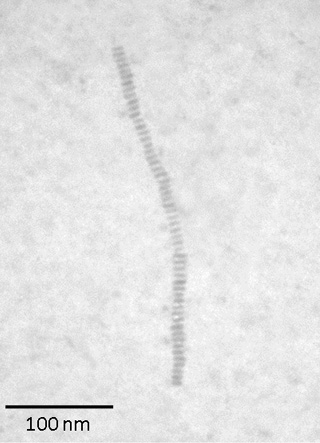This image is a highly magnified photograph captured through a microscope, displaying a white and grayish background with various large gray spots, most likely from light being projected to enhance the visibility of the subject. In the center of the image, a worm-like creature composed of dark gray nubs is depicted stretching vertically from the top to the bottom. Accompanying these nubs are smaller, darker gray dots and dashes aligned in a row. The bottom left corner of the image features a black horizontal line accompanied by text that reads "100 nm," indicating the scale of measurement.